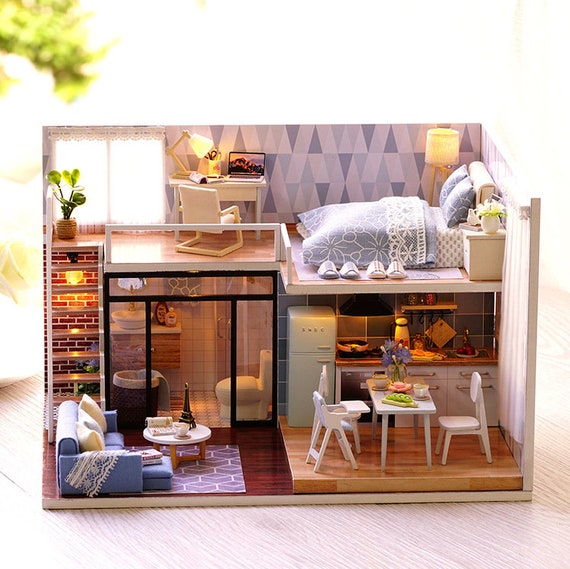This image depicts a highly detailed 3D model representation of a loft-style dollhouse. The dollhouse, placed on a brown wooden surface, provides a comprehensive view of both its upper and lower levels. Constructed in a landscape view within a portrait orientation background, the model features intricate elements that recreate a cozy, livable space in miniature form, ideal for children's imaginative play.

The lower level of the loft showcases a warm and inviting living area with darker brown hardwood floors. Dominating the space is a light blue sectional couch, complemented by a white coffee table with tan legs, resting on a light blue rug patterned with 3D squares. Adjacent to the living area is the kitchen, which slightly elevates on a lighter wood-stained floor. The kitchen is equipped with a white dining table that seats two regular chairs and a high chair for a baby. The table is set with a cutting board of green tomatoes, blue flowers in a vase, two coffee cups on saucers, and a small pink edible item. The kitchen features white cabinets and a range of appliances: a refrigerator to the left, a two-burner stove with a pan, counter space holding another cutting board and a tall jar, a sink area, and shelves stocked with jars.

Ascending a set of white stairs from the living area leads to the upper level, which houses a bedroom and a small office space. The bedroom is furnished with a bed adorned with a light blue and white bedspread, blue pillows, and slippers beside it. A nightstand holds a lamp with a lampshade, a book, and flowers. The upper level maintains the hardwood flooring from downstairs. The office area includes a white desk with a desk lamp and a laptop, complete with a white chair. Above the stairs, a plant in a vase adds a touch of greenery beside a window draped with a light curtain.

Overall, the model's attention to detail, from the blue pyramid-patterned wallpaper to the miniature household items, emphasizes the realism and photographic representationalism style, making it a captivating piece for both children and adults alike.